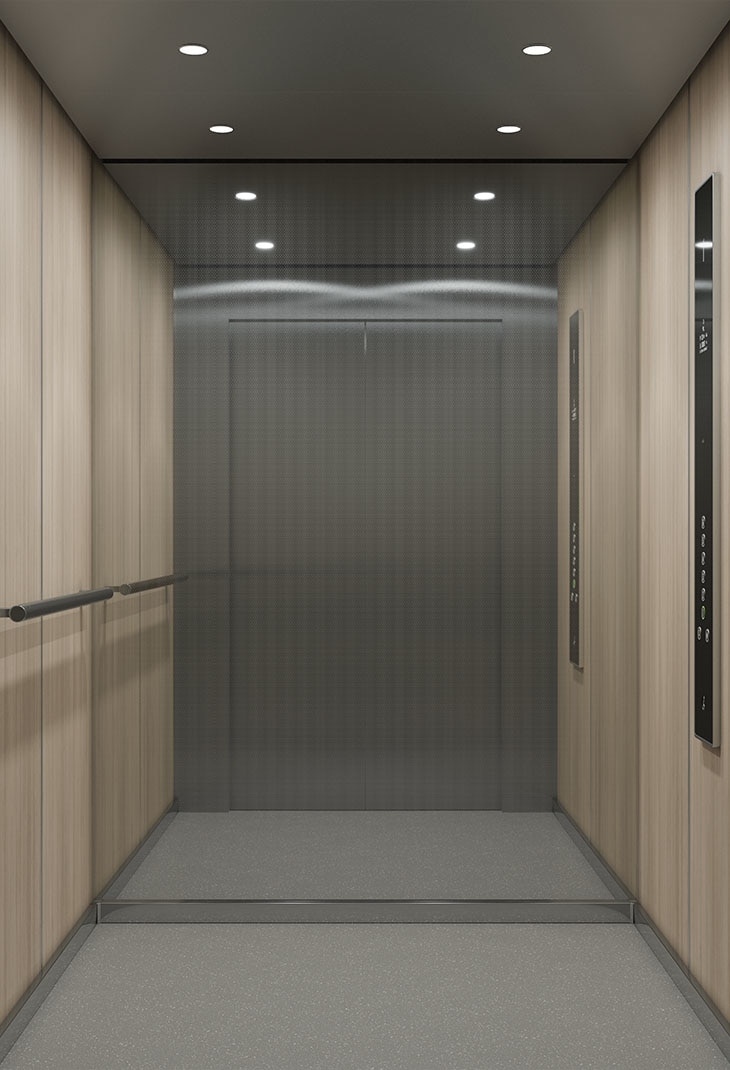This is an image showcasing the interior of a spacious, sophisticated elevator. The vertical, rectangular photo reveals a large, gray metal door at the end, paired with light beige walls. The beige walls host modern features, including a sleek, long silver panel on the right side with buttons that suggest multiple floor selections and additional controls, likely for open, close, and emergency functions. Above, the ceiling is elegantly designed with circular lights, numbering four equally spaced lamps that cast a warm glow over the elevator's interior. A wide mirror on the back wall reflects the hallway, enhancing the sense of spaciousness. On the left side, a silver handrail is present for support, set against the pale wood paneling, which matches the right side's modern decor. The floor is a subtle gray carpet or linoleum, complementing the overall design and creating a refined atmosphere within this upscale elevator.